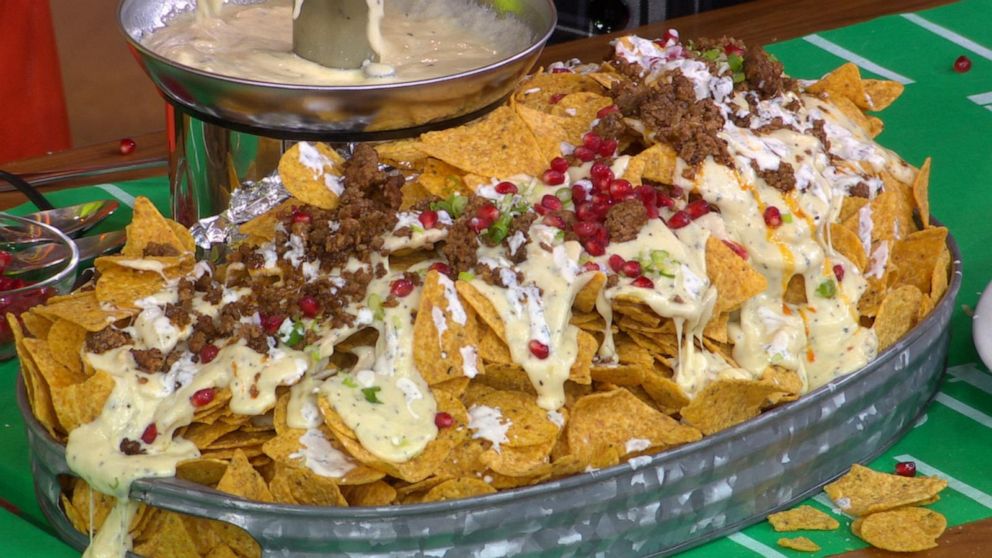The image shows an expansive, oval-shaped metal serving platter filled with golden tortilla chips. These chips are loaded with various toppings, creating a vibrant and mouth-watering display. They are generously covered in melted cheese and dollops of sour cream, complemented by savory ground beef and red beans scattered throughout. Thin green slices, possibly chives or jalapenos, add a touch of color and freshness to the dish. The platter is placed on a green table runner with white lines, resembling a football field, indicative of a sports-themed setup. In the background, a silver bowl containing more of the cheesy topping can also be seen, suggesting it’s a popular dip served alongside the nachos. Some chips have tumbled off the platter onto the table runner, enhancing the casual, indulgent atmosphere of the scene.